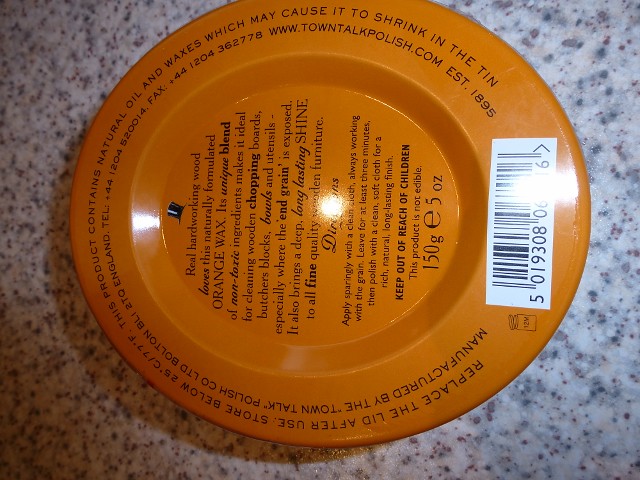The image displays the orange circular lid of a container of orange wax, set horizontally on a speckled granite background. Text on the lid, which is rotated 90 degrees to the left, provides detailed product information and instructions. In black font, it states: "Real Hardworking Wood loves this naturally formulated orange wax. Its unique blend of non-toxic ingredients makes it ideal for cleaning wooden chopping boards, butcher blocks, bowls, and utensils, especially where the end grain is exposed. It also brings a deep, long-lasting shine to all fine quality wooden furniture. Apply sparingly with a clean cloth, always working with the grain. Leave for at least 3 minutes, then polish with a clean, soft cloth for a rich, natural, long-lasting finish. Keep out of reach of children. This product is not edible. 150 grams (5 ounces)." Around the edge of the lid, there's text including storage instructions, manufacturer details, and contact information: "Replace the lid after use. Store below 25 degrees Celsius or 77 degrees Fahrenheit. This product contains natural oils and waxes which may cause it to shrink in the tin. Manufactured by Town Talk Polish, QLTD, Bolton, BLL, 2TQ, England. TEL: +441204520014, FAX: +441204362778, www.towntalkpolish.com, Est. 1895." Additionally, a white barcode is placed near the bottom of the container. The lid sits on a light grey and white speckled granite surface, adding a refined touch to the presentation.